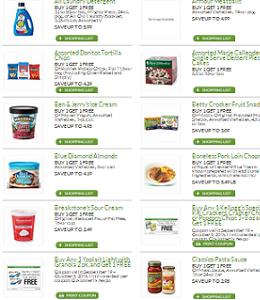An image displays a low-resolution promotional chart featuring various food items from a store, arranged in two columns with six items each. Each item is accompanied by an image on the left and descriptive text on the right. The titles of the items are highlighted in green, followed by black text detailing the offers, which are all "Buy One, Get One Free." Below each section, there is a green button.

1. Detergent
2. Ben & Jerry's Ice Cream - Buy Two, Get One Free
3. Blue Diamond Almonds - Buy One, Get One Free
4. Breakstone's Sour Cream - Buy One, Get One Free (Red carton and tube packaging)
5. Boneless Pork Loin - Buy One, Get One Free
6. Pasta Sauce - Buy One, Get One Free (Two cans: one red and one white)
7. Kellogg's Cereal - Buy One, Get One Free
8. Marie Callender's Entrees - Buy One, Get One Free

This visually cluttered chart is intended to advertise multiple "Buy One, Get One Free" deals on various items ranging from ice cream and almonds to sour cream, pork loin, pasta sauce, and other grocery products.